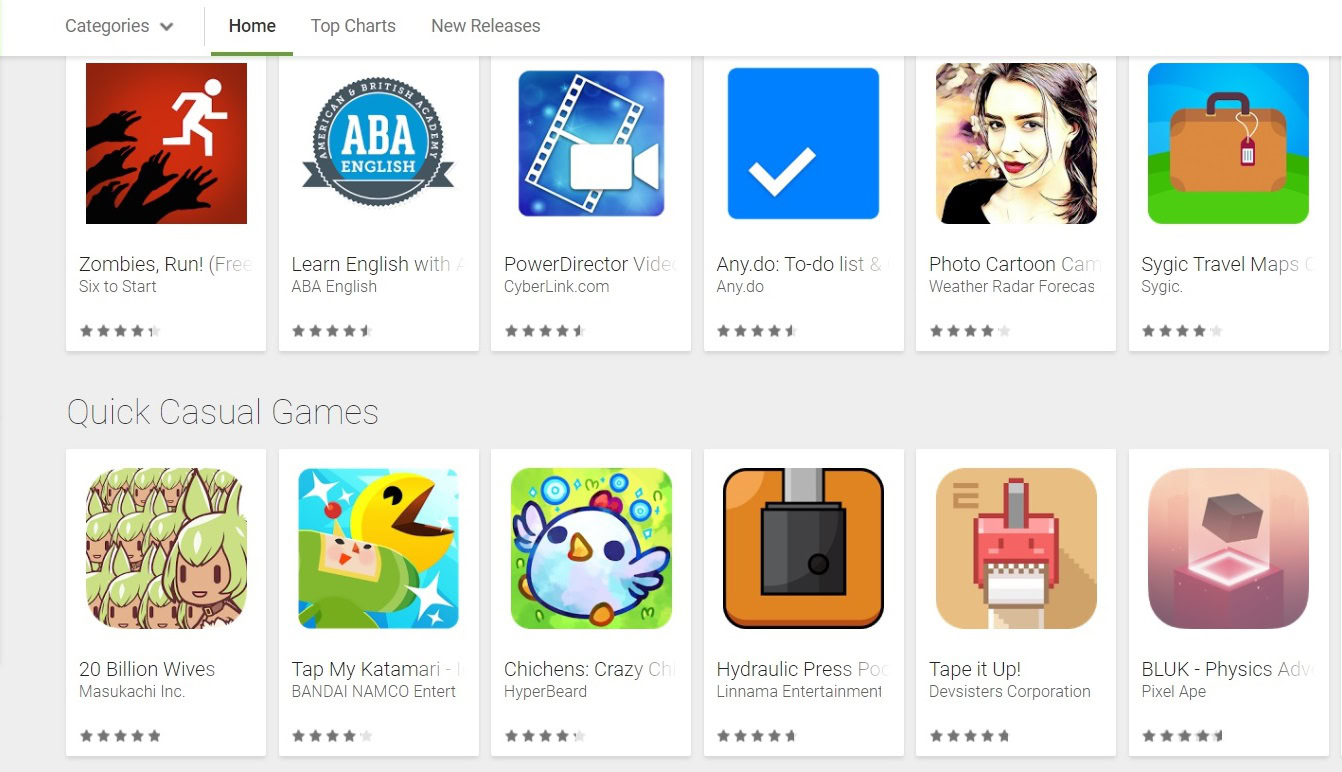The image is a screenshot of a website or app store displaying a variety of games and apps available for download. The interface includes navigation options at the top, labeled "Categories," "Home," "Top Charts," and "New Releases," with "Home" selected and highlighted in green. 

The main section shows five apps with ratings ranging from four to five stars:

1. **Zombie Run Free**: The icon features a white stickman running away from black zombie hands. The tagline reads "Free six to start."
2. **ABA English**: The icon is a circle with a ribbon and the text "American and British Academy." It promotes learning with ABA English.
3. **PowerDirector**: The icon consists of a blue square with a vintage film reel and camera, labeled "video cyberlink.com."
4. **Any.do To Do List**: The icon is a simple blue square with a white checkmark. The visible text reads "any dot do to do list," likely referring to a task management app.
5. **Photo Cartoon**: This app's icon portrays a cartoonized woman and is labeled "caricature." However, the text mentions "Weather Radar," suggesting possible mislabeling.

Further down, the section for "Quick Casual Games" showcases:

1. **20 Billion Wives**: Featuring an anime character with green hair and ears, from Masukachi Inc.
2. **Tap My Katamari**: An icon with an old-style robot and Pac-Man, by Bandai Namco Entertainment, though labeled as "Enter Samsung Entertainment."
3. **Chichens**: A cartoon chicken surrounded by various symbols, from HyperBeard.
4. **Hydraulic Press**: The icon appears to show an orange square within a black square with a silver insertion, from Lenama Entertainment.
5. **Tape it Up**: The icon resembles a cross between a tape dispenser and a wall-mounted fire alarm, created by DevSisters Corporation.
6. **BLUK**: Depicted by a black cube hovering over a white spotlight on a red square, from Pixel Ape.

Overall, the screenshot represents a platform offering a range of games and applications, although the specific website or application name is unclear from the image.